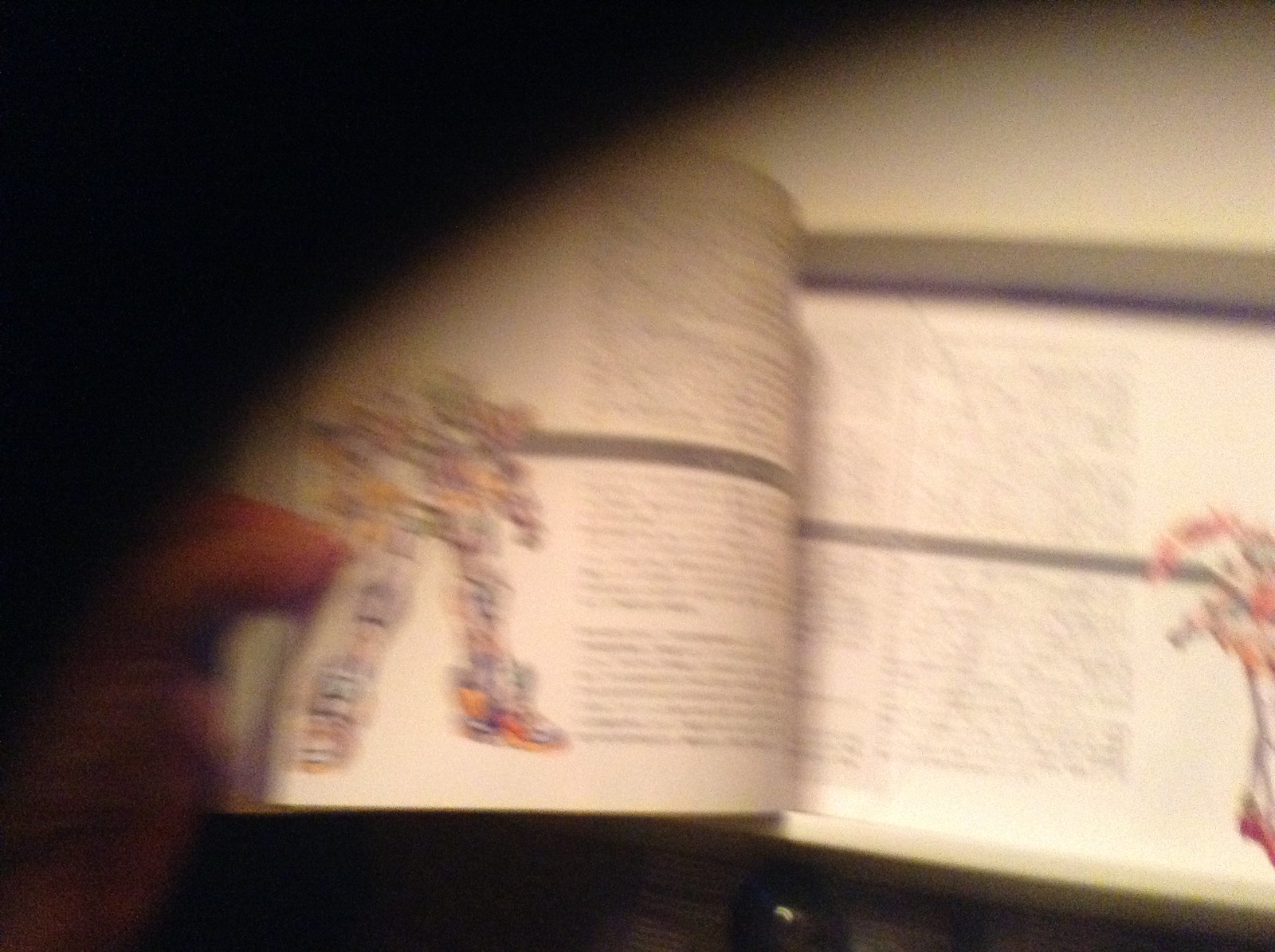This image captures an overhead, first-person perspective of an individual opening a book. The shot appears to be taken as if the camera is mounted on the person's head or possibly integrated into a pair of glasses, providing an immersive viewpoint. The person's left hand is visible, gripping the edge of the book, with their forefinger and thumb prominently appearing in the bottom right corner of the frame. The image is quite blurry, obscuring the book's title and the text within. However, the left page features a vividly colored drawing of a transformer-style robot character, distinct yet not identifiable as any specific cartoon character. The artistic rendering suggests a mechanical, robotic figure typical of the transformer genre.